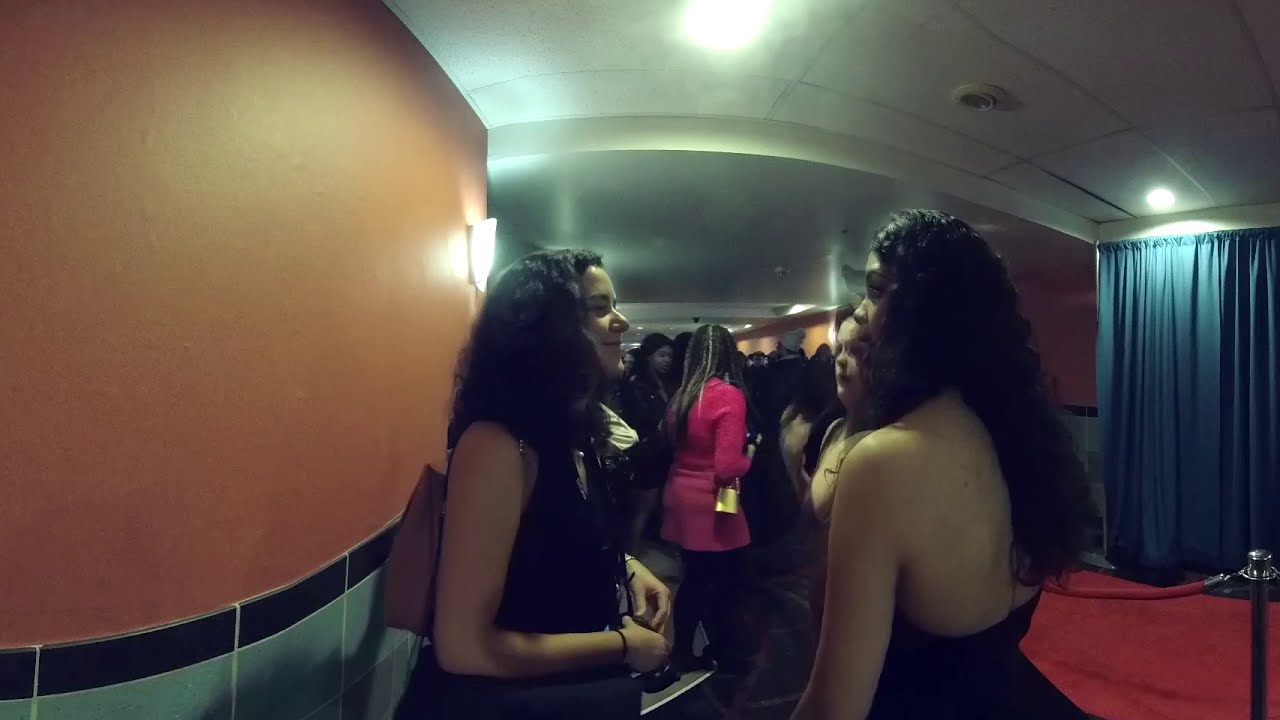In an indoor setting, possibly the entryway of a nightclub or a concert venue, a group of younger women are standing behind a red rope barrier, indicating they're waiting to get into an event. The scene has a somewhat curved panoramic distortion. On the left side of the image, the wall is painted orange and adorned with ceramic tiles in brown and gray, while on the right, a blue curtain hangs from the ceiling, illuminated by a circular light emitting a bluish glow. Another light directly above the group casts a white light with a green outline over the area. The floor here is covered in red carpet.

At the forefront, a young woman in a black dress stands with her back to the viewer, her long black hair cascading down her back. She is looking to her left at another woman who is smiling. This second woman is wearing a dress that covers her shoulder and has her arms raised in front of her stomach. Between them, another woman is walking in the opposite direction, dressed in a long-sleeved pink shirt and carrying a gold purse. The scene captures the anticipation and excitement of the women who are dressed up and waiting to enter a lively event.